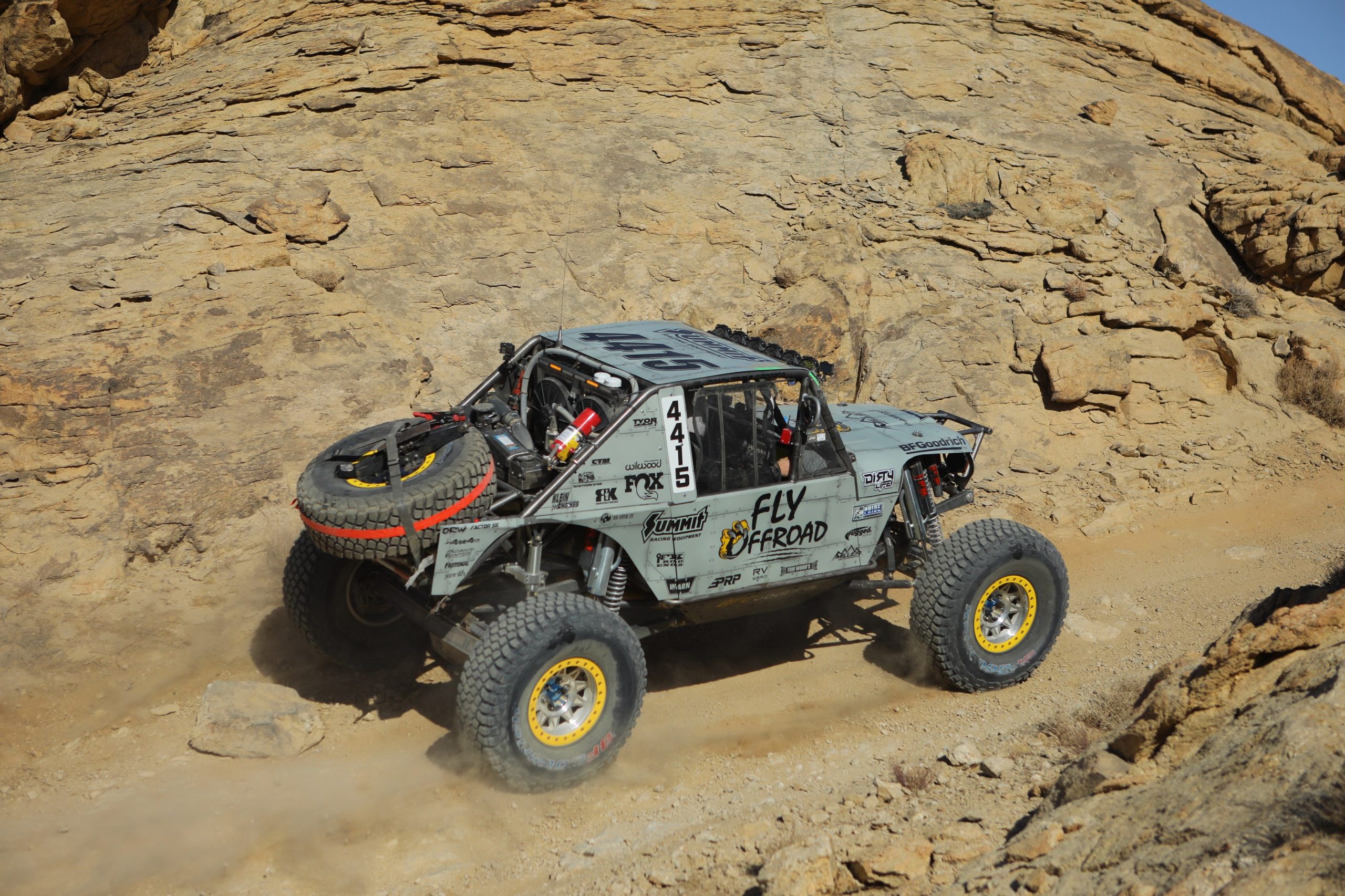The image showcases a rugged, grey monster truck, specifically designed for off-road racing, navigating a dusty dirt path in a desert-like, rocky environment. The elevated body of the truck flaunts exposed big black tires with yellow rims, ensuring it can tackle the toughest terrains. Adorned with numerous sponsor decals, one prominent label reads "Fly Off-Road" on the side, and the race number "4415" is visibly marked downward near the window and on the roof. Additional racing equipment includes a massive spare tire with a red strap and an attached jack, along with a red fire extinguisher for emergencies. This powerful vehicle is equipped with a roll cage for driver and passenger safety, and large shocks are visible. The background features craggy rock formations in light browns and tans, with clouds of dust rising from the moving truck's rear wheels, emphasizing its dynamic motion.